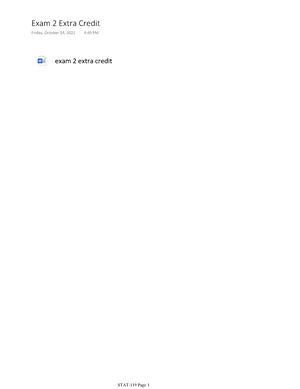A screenshot captures a predominantly white interface, most likely from a digital device like a smartphone or computer. The central focus of the image is black text that reads "Exam 2 Extra Credits," suggesting an academic context such as a school or university. This text might be part of a reminder or notification about an upcoming opportunity for extra credit related to an exam. Below this main text, there is a smaller time indicator displaying "4:XX PM" (the exact minute is indiscernible), which likely signifies the scheduled time for the extra credit exam or assignment deadline. Additionally, a small blue icon accompanies this information, reinforcing the importance or categorization of the event. At the very bottom of the screenshot, more text appears, albeit in a minuscule font, rendering it barely legible. It seems to reference "Page 1," which could indicate pagination or a section of a document. Overall, the screenshot lacks intricate details but clearly pertains to a scholastic reminder involving an extra credit opportunity for Exam 2.